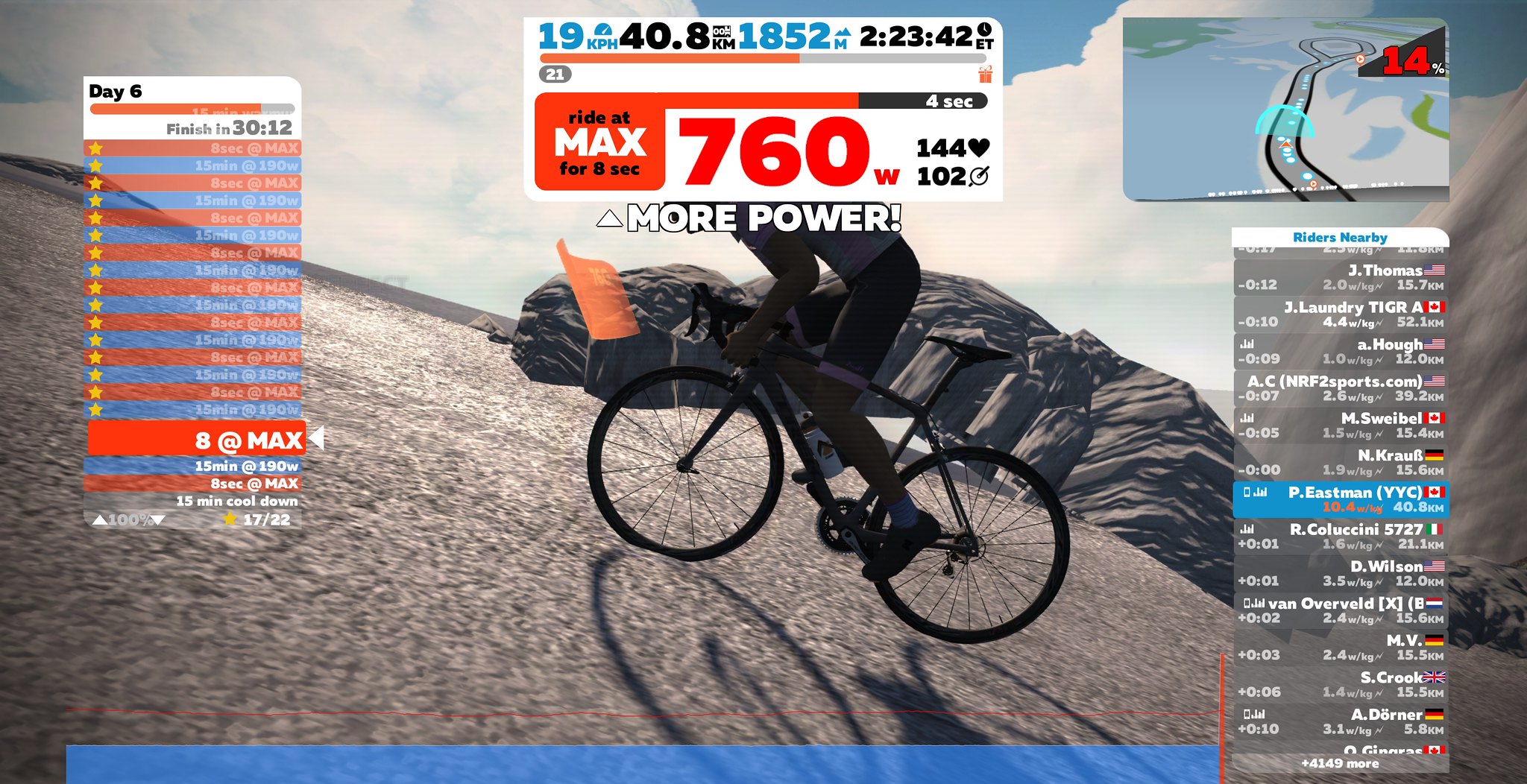This image appears to be a screenshot taken from a video game that simulates a biking experience. The scene shows a 3D-modeled person riding a bicycle uphill against inorganic-looking mountain terrain, which includes synthetic rock formations and a sky with clouds. The graphics appear somewhat low-quality, with awkward lighting and texturing on the rocks.

Overlaying the image is a detailed digital heads-up display (HUD) providing extensive information pertinent to the biker's performance. On the left, there's a panel indicating the day as "Day Six" and showing a countdown timer indicating the biker needs to finish within the next 30 minutes and 12 seconds. This panel also shows the rider's rank among others. Above the biker, there's a directive in a rounded white rectangle urging the rider to "ride at max for eight seconds" to achieve a power output of 760 watts, indicated by "760 W" in large red letters on a white background. Adjacent to this, "144" is displayed next to a heart icon, signifying the rider's heart rate, and "102" is displayed, potentially indicating time or another performance metric.

In the top right corner, a map shows the biker's progress as 14% complete, with additional information about nearby riders, including their countries of origin. This image gives a comprehensive view of various fitness and performance stats for virtual biking, suggesting the game integrates physical activity with competitive and fitness-tracking elements.